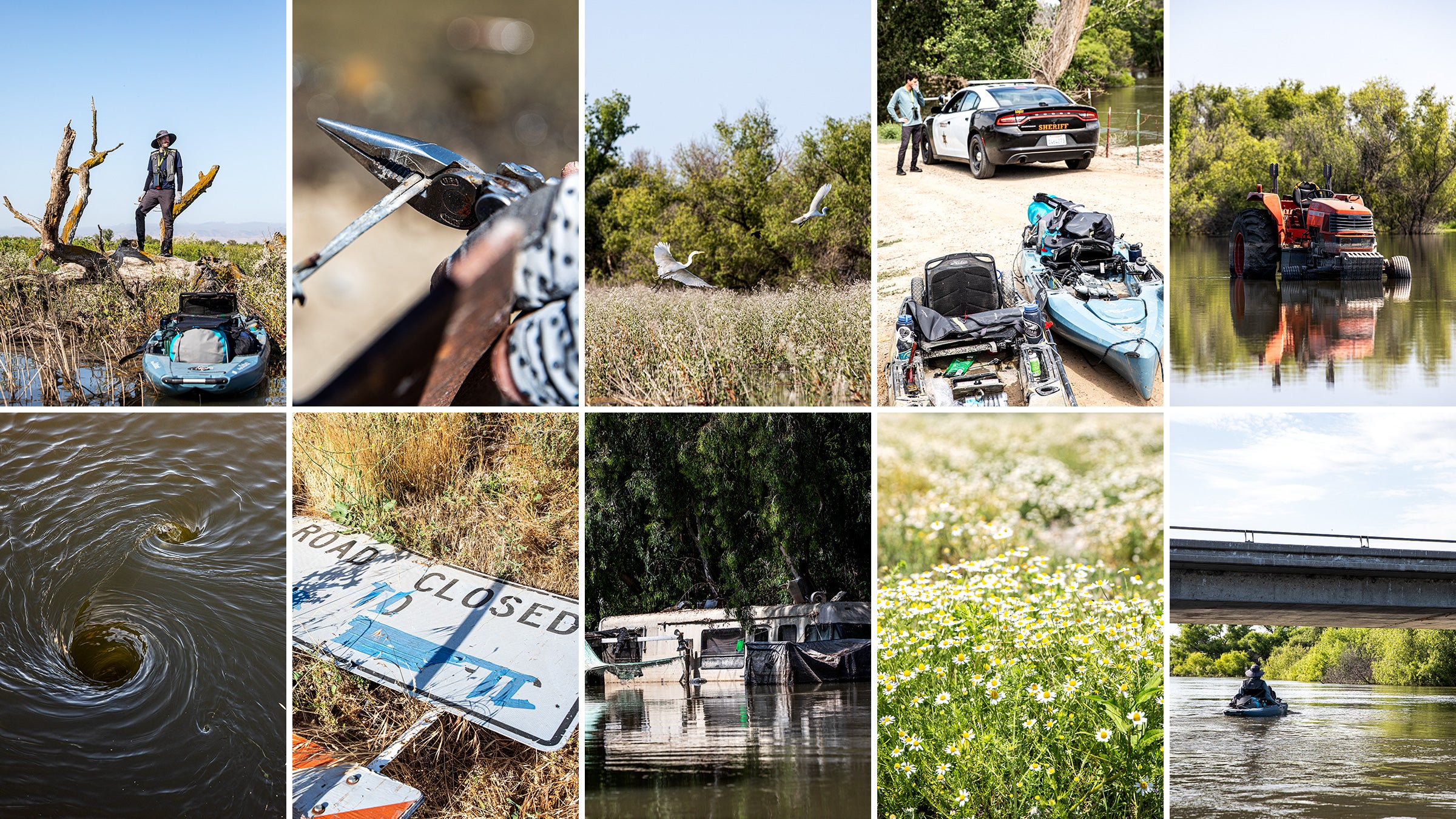The image is a collage of ten outdoor photographs, arranged in two rows of five. Each photograph captures a scene related to a flood's aftermath. 

In the upper left corner, a man stands on the bank of a creek, with his right knee bent and his left leg straight. A kayak is tied up near the water, surrounded by dead trees and rocks. To his right, a person uses needle-nose pliers to cut barbed wire. Further to the right, two crane-like birds take flight from a marshy area under a light blue sky. The next image features a police car in the background with kayaks in the foreground. At the very end of the top row, a large red tractor is submerged up to its tires in floodwater.

The bottom left corner showcases two whirlpools in water, indicating strong currents. Next to it, a fallen street sign reading "Road Closed" lies in the grass, partially covered by blue paint or tape. The following picture shows a mobile home or motorhome half-submerged in water, with trees in the background. The fourth image along the bottom row depicts a field of green grass dotted with small white flowers, resembling daisies. Finally, in the lower right corner, a small boat or kayak navigates a river under a bridge, suggesting high water levels.